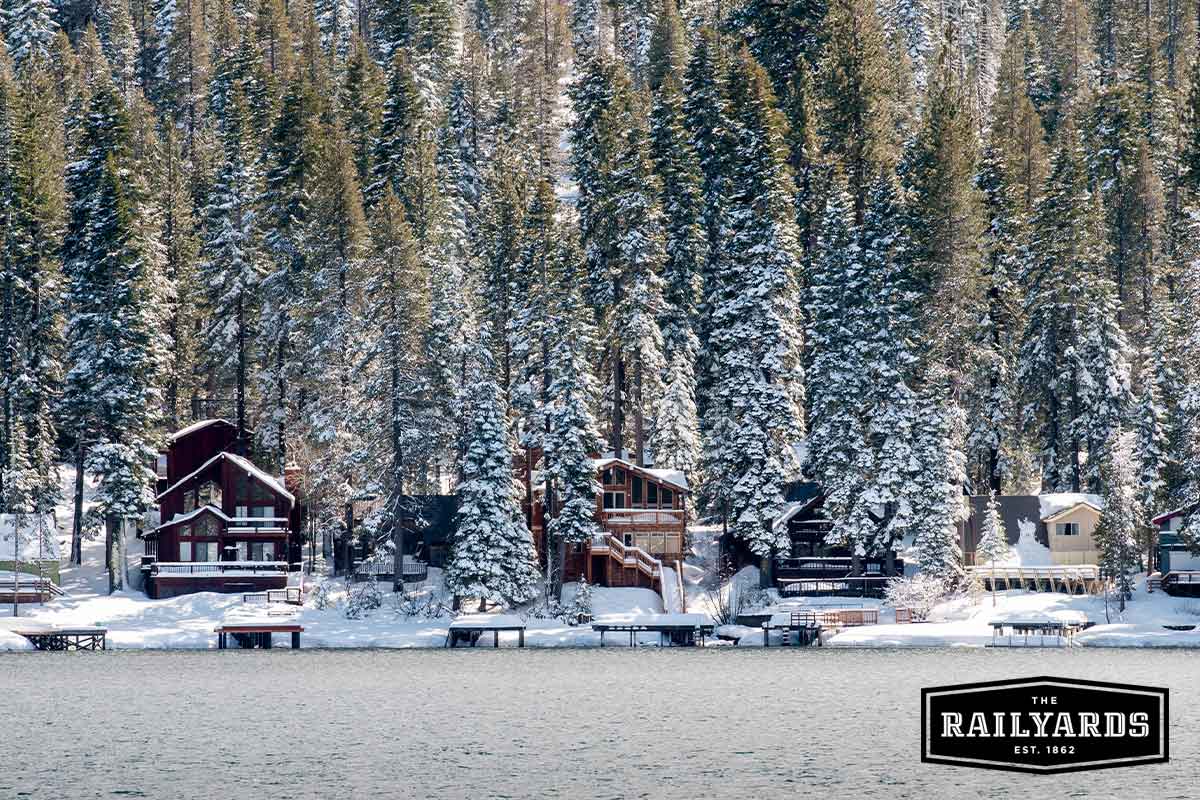This photograph captures a serene winter scene at a high-end resort community situated along the shoreline of a peaceful lake. The opposite shore is adorned with four to five luxurious ski lodges or residences, most of which are three stories tall, with one or two being two stories tall. These homes, characterized by extensive use of glass and clean architectural lines, boast private docks and piers extending into the calm water. Enveloped in a thick blanket of snow, the homes exude a cozy and inviting atmosphere. Nestled within a dense forest of tall, snow-capped pine trees, the lodges are set against the backdrop of towering, snowy mountains. The entire landscape glistens under the bright sunlight. Notably, the bottom right corner features a logo that reads "The Rail Yards, Established 1862," indicating that this picturesque scene is part of a historic resort community.